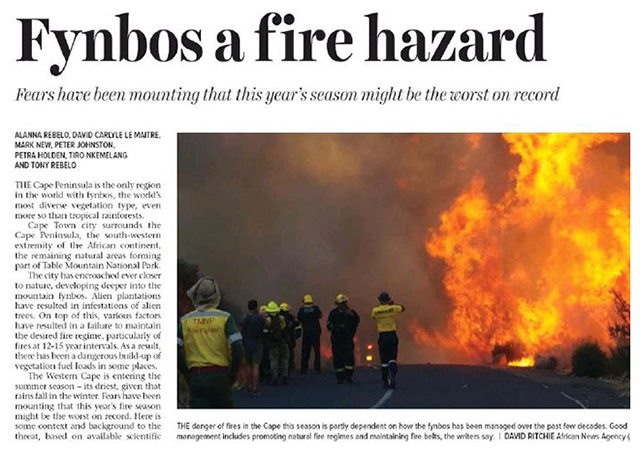Screenshot from a newspaper article. The headline in large black text reads: "FinBoss a Fire Hazard." The subtext underneath states: "Fears have been mounting that this year's season might be the worst on record." To the left, a column of text offers more detail about the situation.

To the right, there is a large, dramatic image showing numerous firefighters in their protective uniforms standing on the left lane of a road. They are intently looking into a blazing fireball with a massive gray plume of smoke rising into the sky on the right-hand side of the road. The fire, towering at about four to five times the height of the firefighters, dominates the scene. In the distance, a red warning light can be seen amidst the chaos. Some firefighters are equipped with helmets, while at least two are not. Their uniforms are primarily bright yellow, and those who lack yellow tops have trousers with reflective strips.